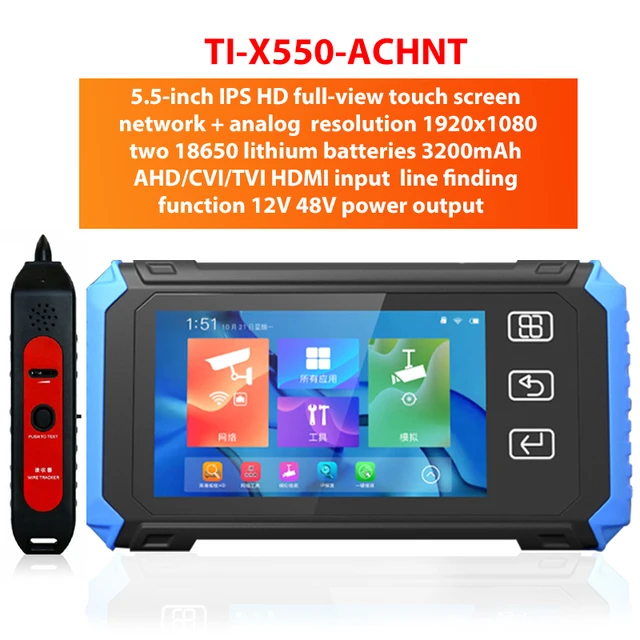This advertisement for the TI-X550-ACHNT prominently features its name in bold red capital letters at the top. Below the title, an ombre rectangular box transitions from a lighter yellow-orange to a darker red-orange on the right. The white text within the box provides detailed specifications: "5.5 inch IPS HD full-view touchscreen network and analog resolution 1920 x 1080, two 18650 lithium batteries with 3200 mAh capacity, AHD/CVI/TVI, HDMI input line finding function, and 12V/48V power output."

The lower segment of the advertisement showcases two distinct devices. To the left, there is an oval black piece of plastic with a red inner oval housing two ports: one oblong, sideways oval, and the other circular. To the right, a smartphone-like device is encased in a black case with light blue edges on the sides. The screen displays a blue, swirly background resembling a Windows interface, adorned with colorful icons including orange, blue, purple, and green. The device's interface also features foreign characters, likely Chinese, suggesting a multilingual capability. Additionally, the unit includes several console buttons on the right side.